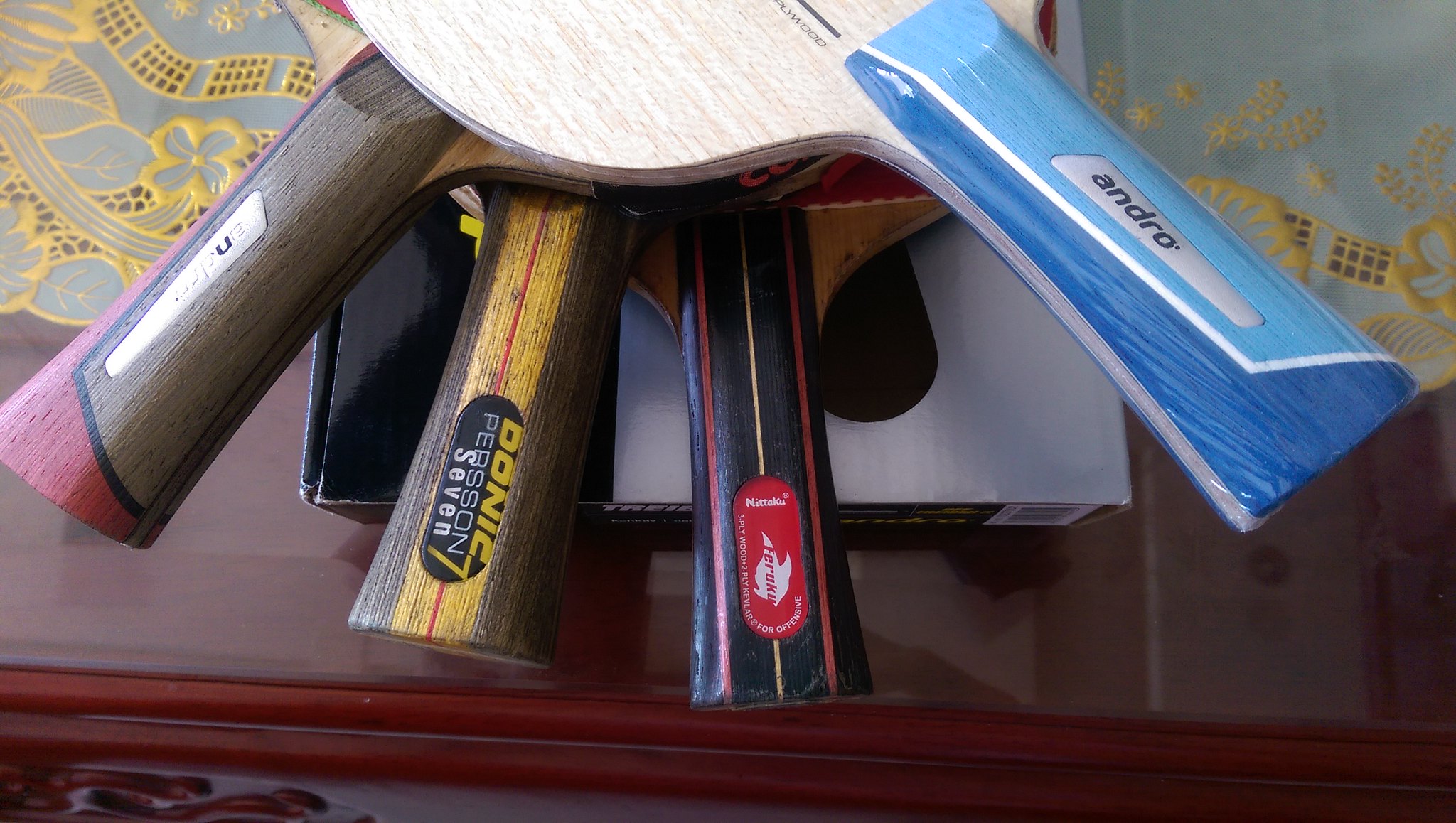In this photograph, we see a vibrant display of high-quality ping-pong paddles meticulously arranged on a mahogany wood surface. There are four paddles in total, each distinguished by its unique design and handle color. The paddle on the top features a light wood whitish color, with a darker blue handle accented by a white and lighter blue strip, and a gray spot labeled "Andro." There's also a paddle with a brown handle and red accents at the bottom left. Another paddle showcases a yellow and red handle with brown edges, while the fourth paddle has a predominantly black handle with red and yellow lines running along its length. These paddles are resting on a box, likely part of the display setup for one of the paddles, enhancing the overall presentation of the equipment.